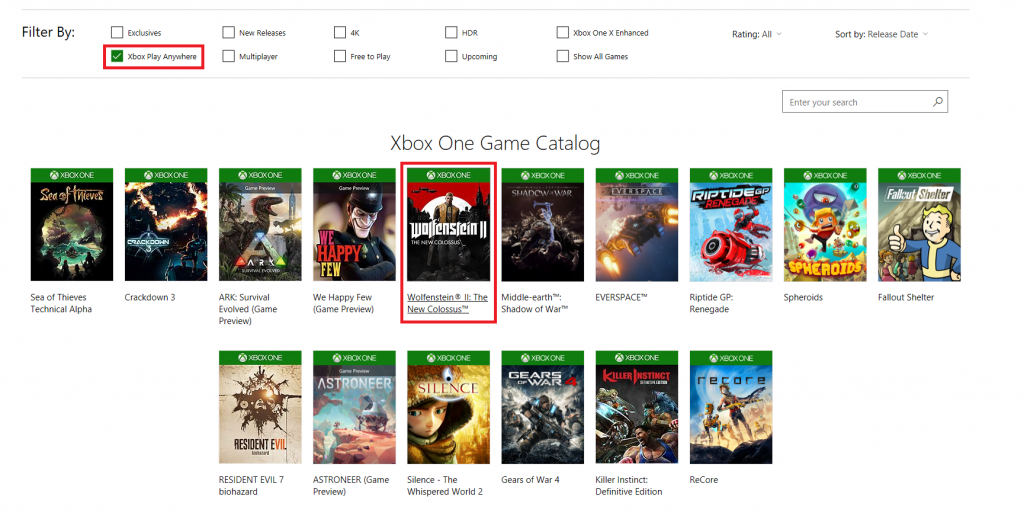This detailed caption elegantly describes the screenshot:

---

**Screenshot Description: Xbox One Game Catalog**

The image captures a detailed view of the Xbox One game catalog interface. At the top, a variety of filter options are visible, organized into two horizontal rows. The filters include categories such as 4K, Free-to-Play, HDR, Upcoming, New Releases, Multiplayer Exclusives, Enhanced, Show All Games, and Ratings. There is also a search bar available for more specific queries.

A red rectangle highlights the active filter, "Xbox Play Anywhere," indicating that this specific filter is currently selected. 

Beneath the filters, the catalog displays a series of game covers. The layout features ten game boxes arranged in two rows at the top and an additional six boxes aligned below, all centered against a white background. Each game cover prominently displays the Xbox One logo set against a green field at the top of the box.

Among the displayed titles, "Wolfenstein II" is highlighted as the selected game. The screenshot is focused on this segment of the interface, with no additional footers or extraneous elements visible.

---

This caption provides a comprehensive and detailed overview of the content shown in the screenshot.